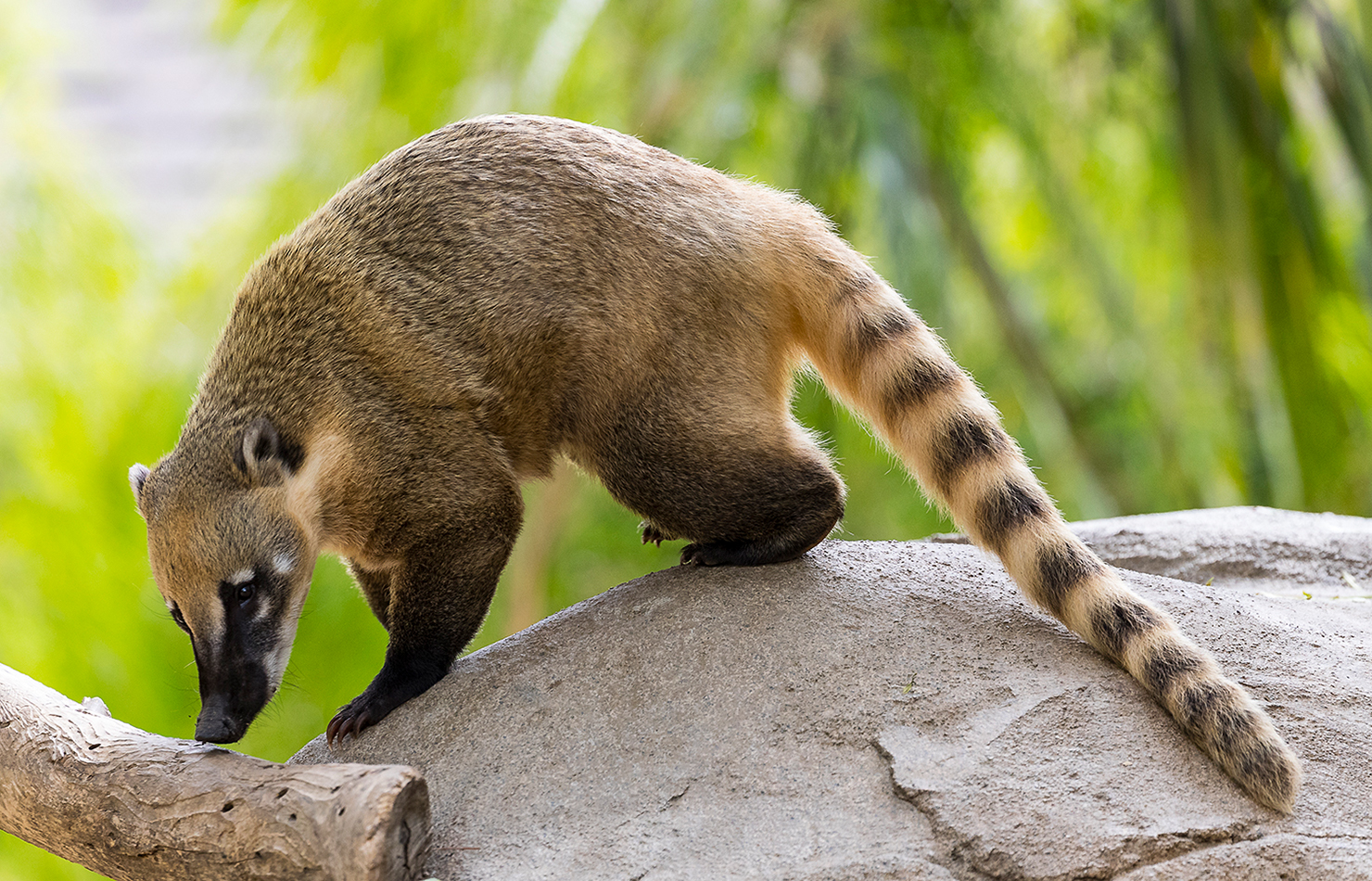In the foreground of the photograph, a small mammal is standing on a large brownish-grey rock that occupies the bottom quarter of the frame. To the left of the mammal, a brownish-grey stick extends out of the frame. The mammal, positioned towards the center left of the frame, has a distinctive and exotic appearance reminiscent of a cross between an anteater and a raccoon. It features beige and black striped fur, most prominent on its long, raccoon-like tail that trails off to the bottom right atop the rock. The creature's body is covered in mottled shades of beige and dark grey, curving upwards to the left, leading to its head which is lowered to sniff the stick. The mammal's face is characterized by a long, pointed black nose, black eyes encircled by black and white spots, and small, pointed ears perched just behind the eyes. Its legs and feet are black, equipped with dark brown, sharp claws, suitable for digging. The background is a blurred vista of bright green foliage, adding a sense of depth and natural habitat to the scene.